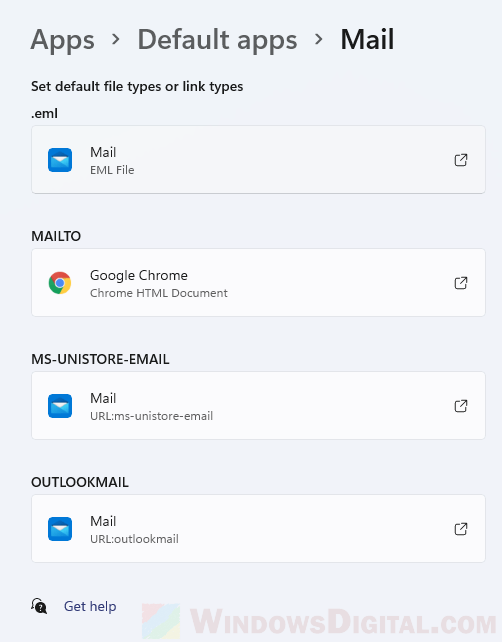The image depicts a subfolder dedicated to managing mail settings within an application. At the very top, the hierarchy is described with the label "Apps" followed by a small arrow leading to "Default Apps," and then another arrow pointing to "Mail." 

Just below that, there is an option labeled "Set default file types or link types." This section is arranged into four distinct subsections, each visually separated by a bold title. 

The first subsection is detailed as follows: it features a bold title ".eml," which is supported by a rectangular region that spans the width of the section. Within this rectangle, there is a small blue mail icon, adjacent to text that reads "Mail" and ".eml file." On the far right side of this rectangle, there is an icon of a square with an arrow pointing outwards, suggesting that interacting with this component will open a new window.

The remaining subsections follow a similar format: they consist of long white rectangles that contain specific icons and descriptions relevant to their function, as well as the square-and-arrow icon which indicates that additional settings or information can be accessed in a new window.